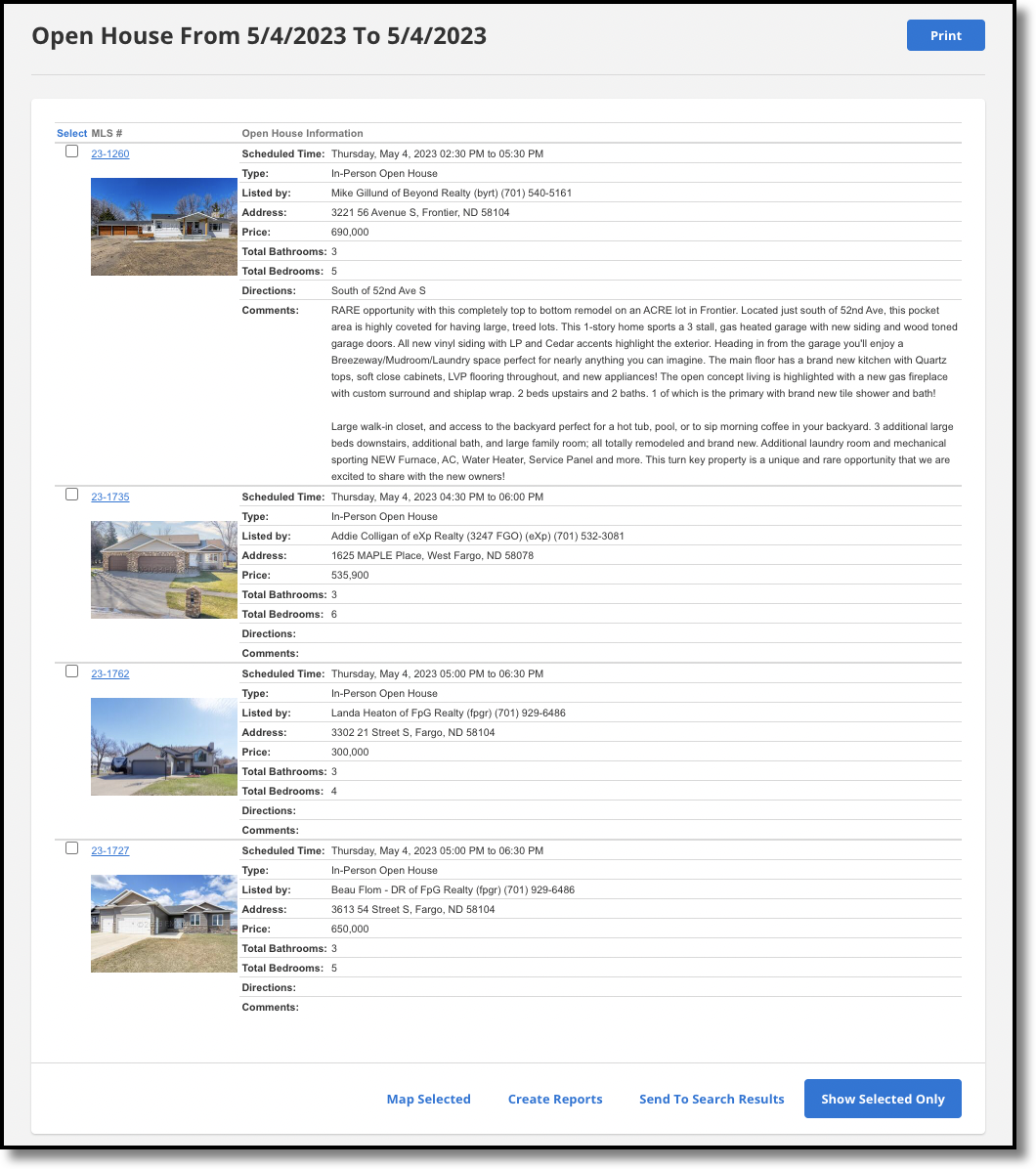Join us for an in-person open house event titled "Michelangelo: Beyond Reality" on Thursday, May 4th, 2023, from 3:00 PM to 5:00 PM at 3221 Southwest Second Avenue. This exquisite property, listed at $169,000, features a spacious 6,000 sq ft living area. 

The home boasts a total value of approximately $133,000 to $145,000, including a large walk-in closet adjacent to a versatile backyard—ideal for installing a hot tub, a pool, or simply enjoying your morning coffee. 

The ground floor includes three expansive bedrooms, an additional bathroom, and a sizable family room, providing ample space for a modern lifestyle. 

Additional amenities include a convenient laundry room and upgraded mechanical systems, including a new air-conditioning unit. Don’t miss this unique opportunity to explore a remarkable home in person. Thank you!